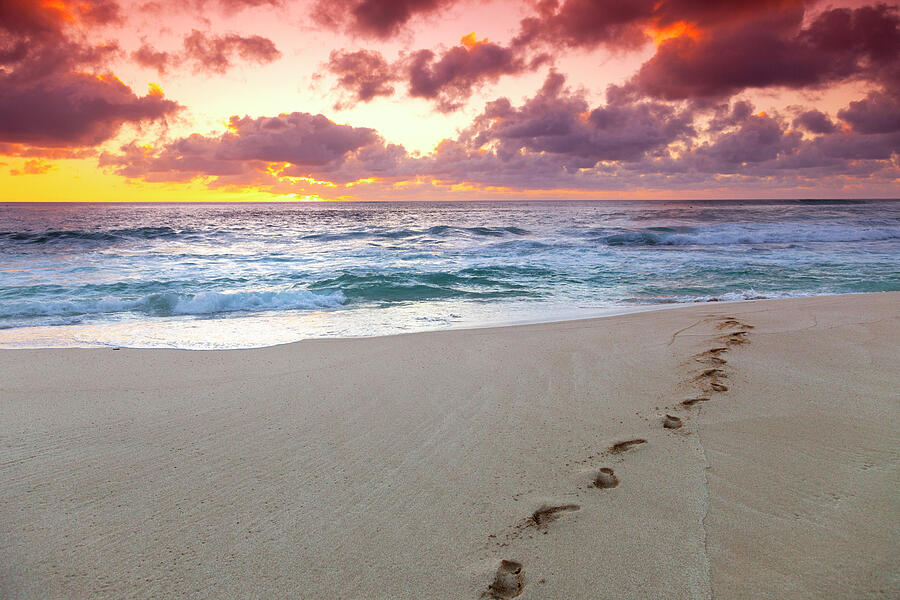The photo captures a serene beach scene with a sandy shore extending towards a calm, blue ocean. A single set of footprints leads from the foreground straight to the water's edge, suggesting a solitary walk. The sky above is a mesmerizing gradient of colors—red, yellow, orange, and peach—indicative of either sunrise or sunset. Light, wispy gray and white clouds float in the sky, adding texture to the horizon. The sand is a light tan to slightly white hue, particularly where the reflective sunlight casts a glow. The ocean is peaceful, with shallow waves gently lapping against the shore, reflecting the golden tones of the sun. There's a sense of quiet and tranquility in the image, as the vibrant, colorful sky meets the calm, blue sea.